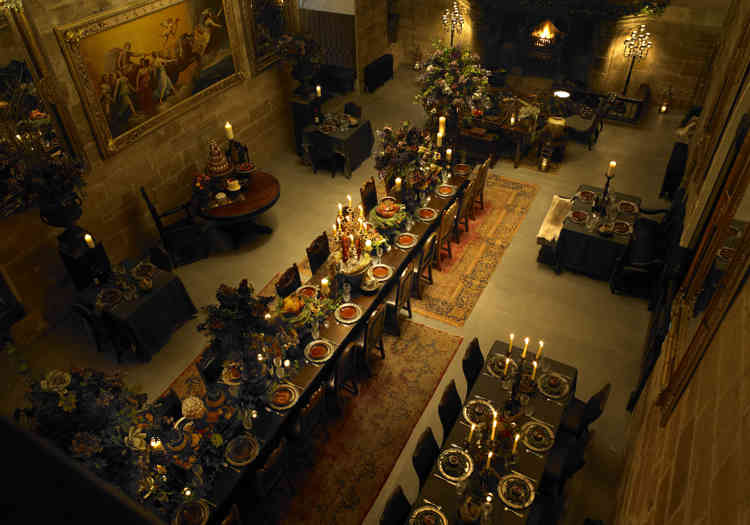The image captures an opulent dining room, reminiscent of an old castle, elegantly adorned for Christmas. Taken from an elevated vantage point, likely the second or third floor, the photograph offers a comprehensive view of the grand room below. Central to the scene is a massive wooden dining table surrounded by approximately 20 high-backed, medieval-style chairs, exuding a regal ambiance. This central table is meticulously arranged with plates of prepared food, candelabras, and large floral bouquets, enhancing the luxurious setting.

To the left of the main table, another lengthy table is set with eight place settings, each accompanied by ornate decorations. Additionally, a smaller table with four place settings, featuring a single candle, is visible above the larger tables. 

Adding to the festive atmosphere, Christmas decorations are tastefully dispersed throughout the room. A small Christmas tree stands atop a wooden table, its presence complemented by other holiday adornments. A striking large painting, framed in gold and depicting men intermingling with angels, graces the wall, further emphasizing the room's majestic and historical character.